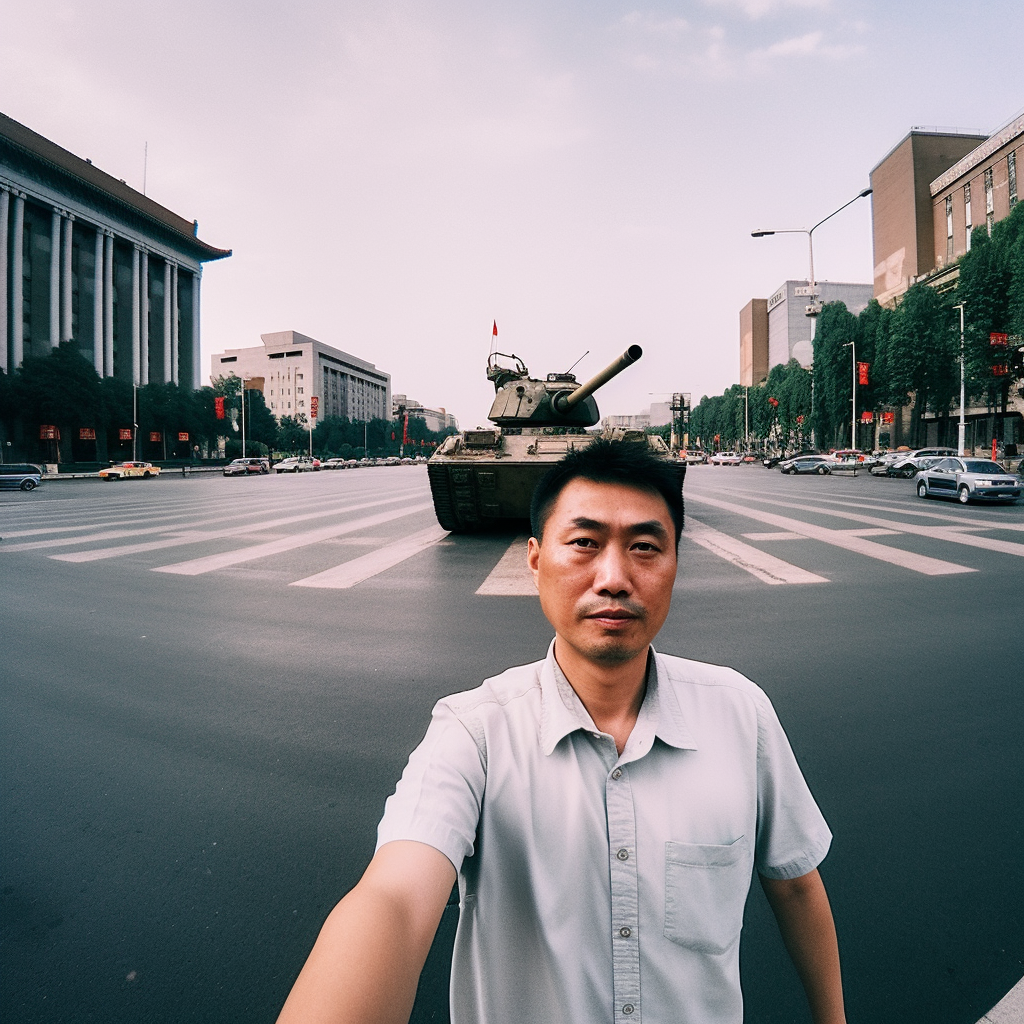In this striking outdoor city scene captured with a photographic style using a wide-angle lens, an Asian man stands in the foreground, appearing serious and somber as he likely takes a selfie with an extended arm. He sports a button-down shirt in either light blue, grey, or beige, with short sleeves and no tie. His short black hair is slightly longer on top, and he has a modest mustache and beard. 

Behind him, dominating the scene is a turreted tank, its gun barrel pointed slightly away from the camera, positioned on a broad crosswalk that spans the middle of a wide street. Flanking the street are parked cars and an assortment of buildings: to the left, a distinctive tall building featuring a pagoda-style roof and grey columns, complemented by street lamps and red banners; to the right, a mix of multi-story brick buildings and a white structure. Both sides of the street are also dotted with green trees, contributing to the urban greenery. The sky overhead is a blend of light grey clouds and patches of blue, adding a subtle atmospheric touch to the photograph. The text on distant signs remains unreadable, maintaining the focus on the poignant juxtaposition of the man and the tank behind him.